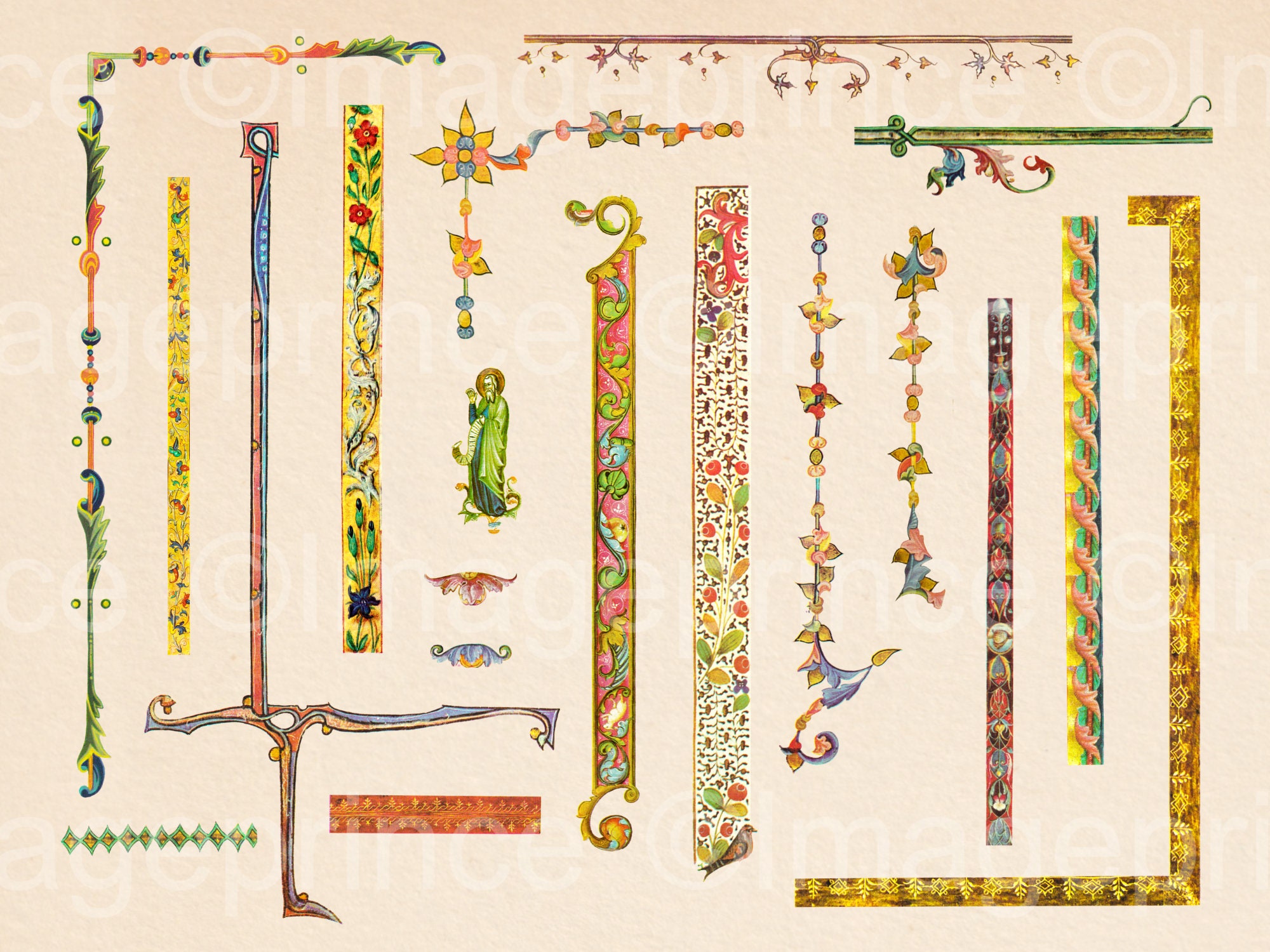The image is an illustrated compilation of various border and bar designs, all set against a light beige background. In the top left corner, there's a border characterized by a floral pattern in greens and oranges, which could be fitting for a book cover. This is followed by a yellow strip adorned with flowers painted in red, green, and white. There's also a pinkish border with more leaf designs, a gold strip with gold leaves, and a solid green border featuring plant motifs.

Toward the center of the image, more colorful and visually interesting bars stand out amidst the repeating patterns. Notably, to the left of these central bars is a small yet distinct illustration of a saint, depicted in classic Christian iconography with long robes and a halo.

Overall, the borders and bars, which primarily run vertically with some bending at 90-degree angles, appear to be intended for lining the edges of pages or book covers, reminiscent of old-style design flourishes. Additionally, a faint watermark, seemingly reading "Image _____" (possibly Image Bounce or Image Prime), is visible throughout the background, blending subtly into the beige backdrop.